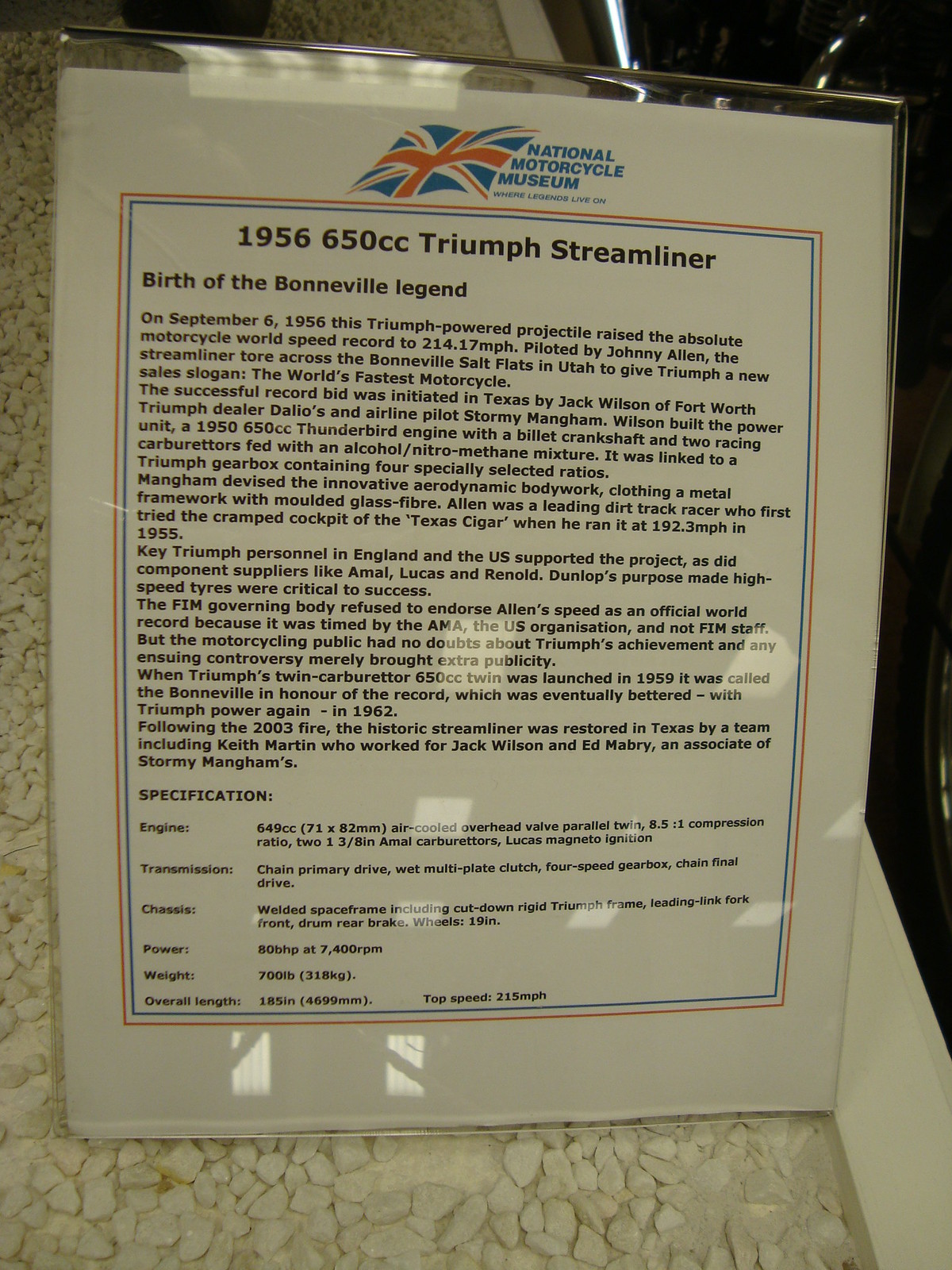The photograph captures an information board from the National Motorcycle Museum, housed within a glass case. The information, printed on white paper, is prominently titled "1956 650CC Triumph Streamliner" in black font, enclosed within a blue and orange rectangle. At the top, the sheet bears the text "National Motorcycle Museum" in blue, alongside a British flag logo. The information provided delves into the birth of the Bonneville legend, recounting the history and notable achievements of the 1956 Triumph Streamliner, including its world speed record of 214 miles per hour. Below the historical narrative, the board details specifications such as engine, transmission, chassis, power, weight, overall length, and top speed. The background of the image features a white, pebble-like wall reminiscent of faux gravel.